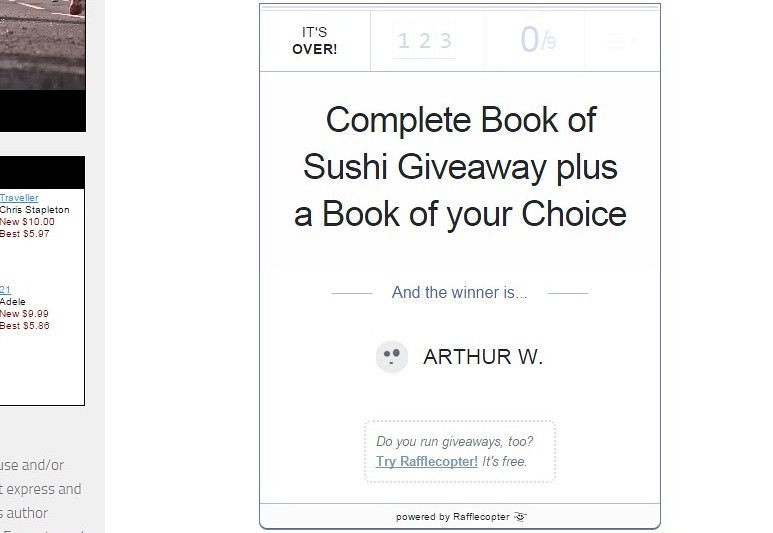The image displays a web page with a rectangular social media post-style announcement on a white background with a gray frame. It declares the conclusion of a "Complete Book of Sushi" giveaway, also offering the winner a book of their choice. At the top of the post, it reads "It's over" followed by the numbers "1, 2, 3, 0, slash, 9." Below that, in bold black text, it announces the winner: "Arthur W.", alongside a simple graphic of a gray, round face with two eyes and a mouth. Further down, within a dotted box, an advertisement prompts viewers with "Do you run giveaways too? Try Rafflecopter. It's free." At the very bottom, an additional note reads "Powered by Rafflecopter," accompanied by a small helicopter icon. The entire layout is more vertical than horizontal, emphasizing its elongated form.